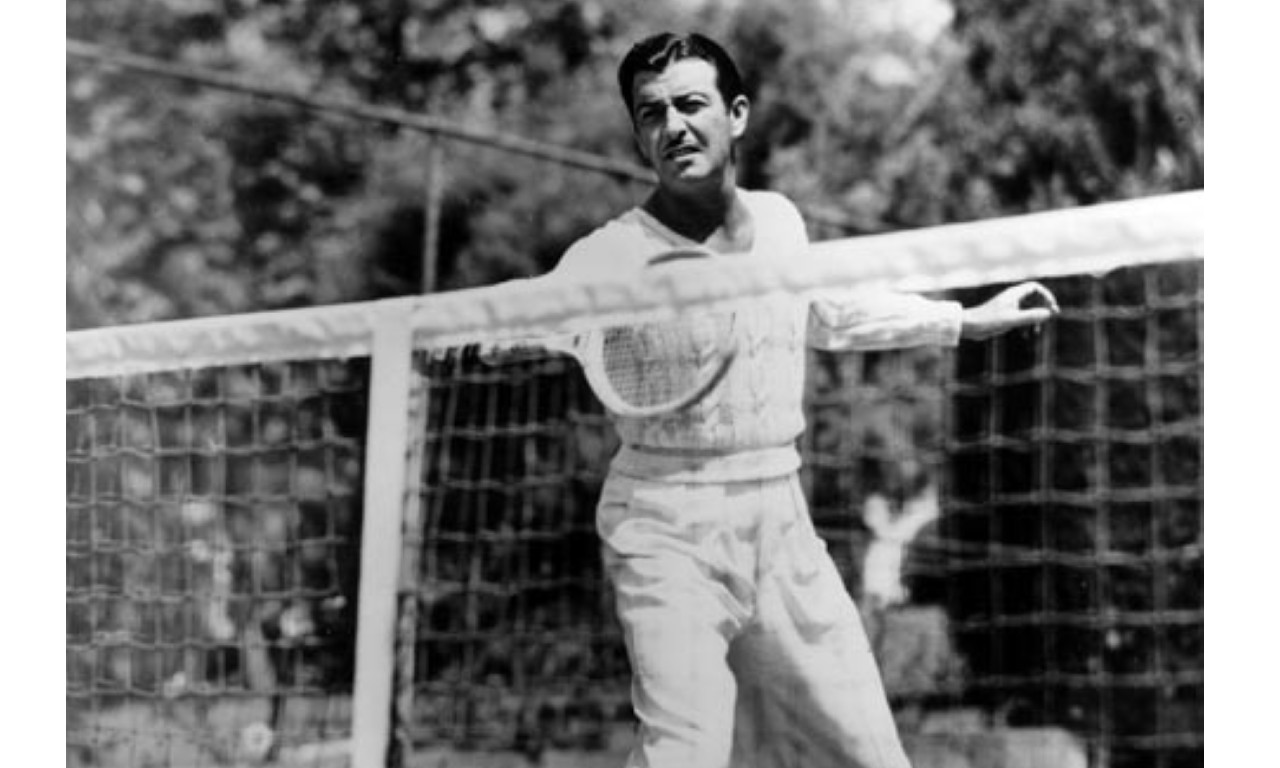In this vintage black and white photograph, a man, identified as possibly the famous actor Clark Gable from the movie *Gone with the Wind*, is captured in the midst of a tennis game. He sports a thick mustache, thick eyebrows, and short dark hair, with a sweater and white slacks typical of the 1920s attire. The man stands at the net of an outdoor tennis court, poised in a backhand position with his right hand gripping the racket while his extended left hand balances him. The court is enclosed by a chain-link fence, beyond which a line of trees is visible. The middle of the net features a strap holding it down. The photograph, showing the details of his pose and surroundings, offers a nostalgic glimpse into a past era of sports and leisure.